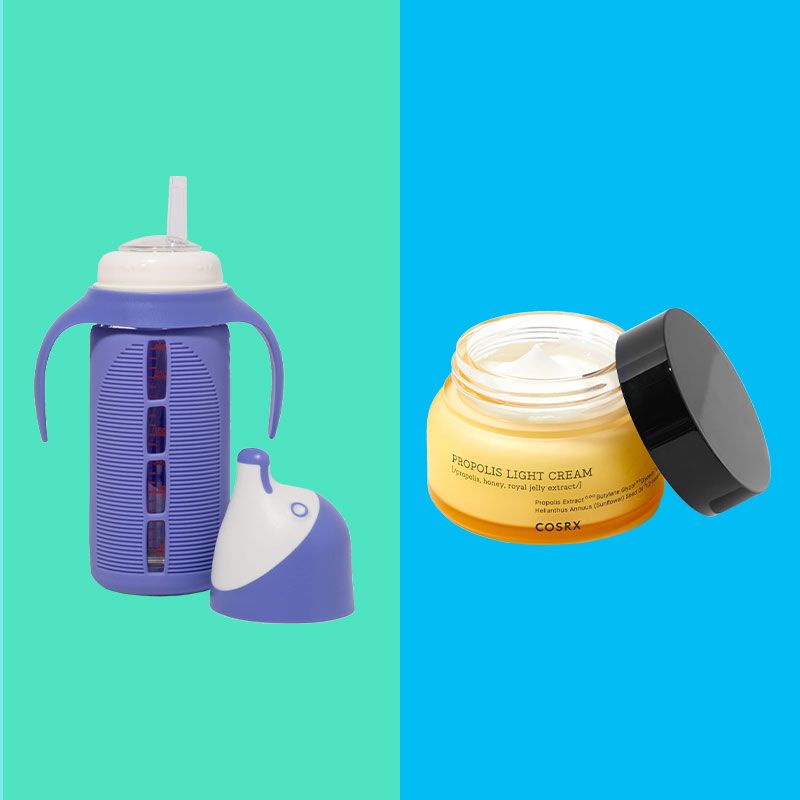The image features two distinct products, each positioned in front of contrasting backgrounds. On the left, there's a toddler sippy bottle situated against a green background. The bottle, made of clear glass, is encased in a purple rubber sleeve with two outward-flaring handles. The sleeve has small windows to show the remaining liquid. It comes with a cap designed like a whimsical penguin head with a white face and purple accents. This cap can be used or removed to expose a sippy spout.

On the right, set against a blue background, is a beauty product—a jar of Propolis Light Cream. The jar itself is made of clear, yellow-tinted glass, revealing the light-colored cream inside. It comes with a sleek black lid, which is leaning against the jar. The cream is intended for facial use, likely as a nighttime skincare treatment.